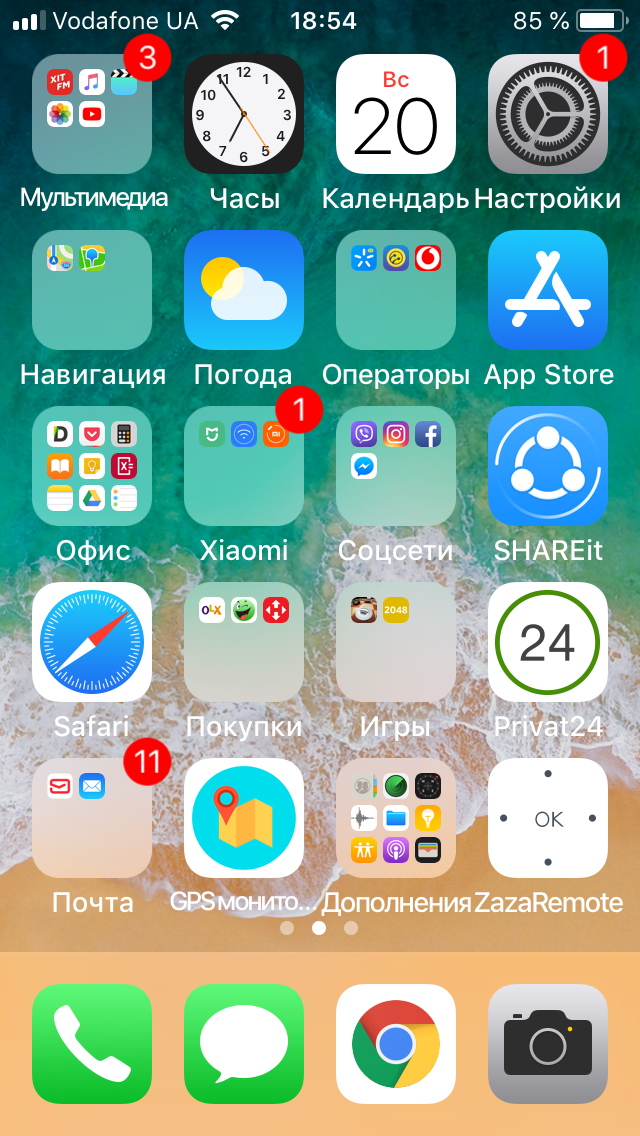This is a detailed caption for the provided image description:

---

Screenshot of a smartphone displaying a mix of various app icons on the home screen. The phone interface is primarily in a non-English language, with only a few elements in English. At the top left corner of the screen, the Wi-Fi signal icon is visible, followed by the text "Vodafone UA.” Next to it is the network signal strength indicator, the time "18:54," and the battery level, which shows "85%." These elements are all displayed in white.

The home screen has five rows of app icons, each varying in color and style. At the very bottom, there are four main icons in the dock: a white telephone on a green background (likely for the phone app), a white speech bubble icon on a green background (messaging app), the Google app icon, and a black camera on a gray background (camera app).

The overall background of the home screen features green, white, and yellow hues that appear to depict an ocean scene. Among the apps, the only readable English labels are for the "App Store" and "Safari." On the bottom right corner of the screen, there is another readable app labeled "Zaza Remote."

---